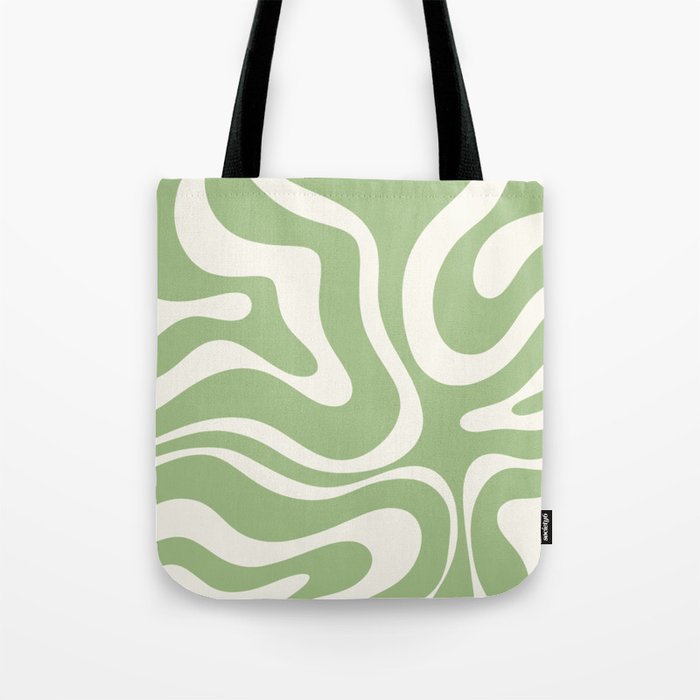The image is a square photograph of a canvas tote bag positioned centrally on a plain white background, resembling a product shot you'd find on an online shopping site. The tote bag displays an abstract, swirly pattern of light green and white, with random lines seamlessly flowing across its surface, reminiscent of a meandering river breaking up the solid green with delicate, white trails. The bag is equipped with long, black handles made of a sturdy material, suitable for carrying over the shoulder. On the bottom right corner of the bag, there is a small black tag featuring some text, presumably the brand name, though it is too small to read clearly. The overall color palette of the image includes black, white, and light green, creating a vibrant yet simple aesthetic for the tote bag, which appears spacious enough to accommodate items like a laptop or groceries.